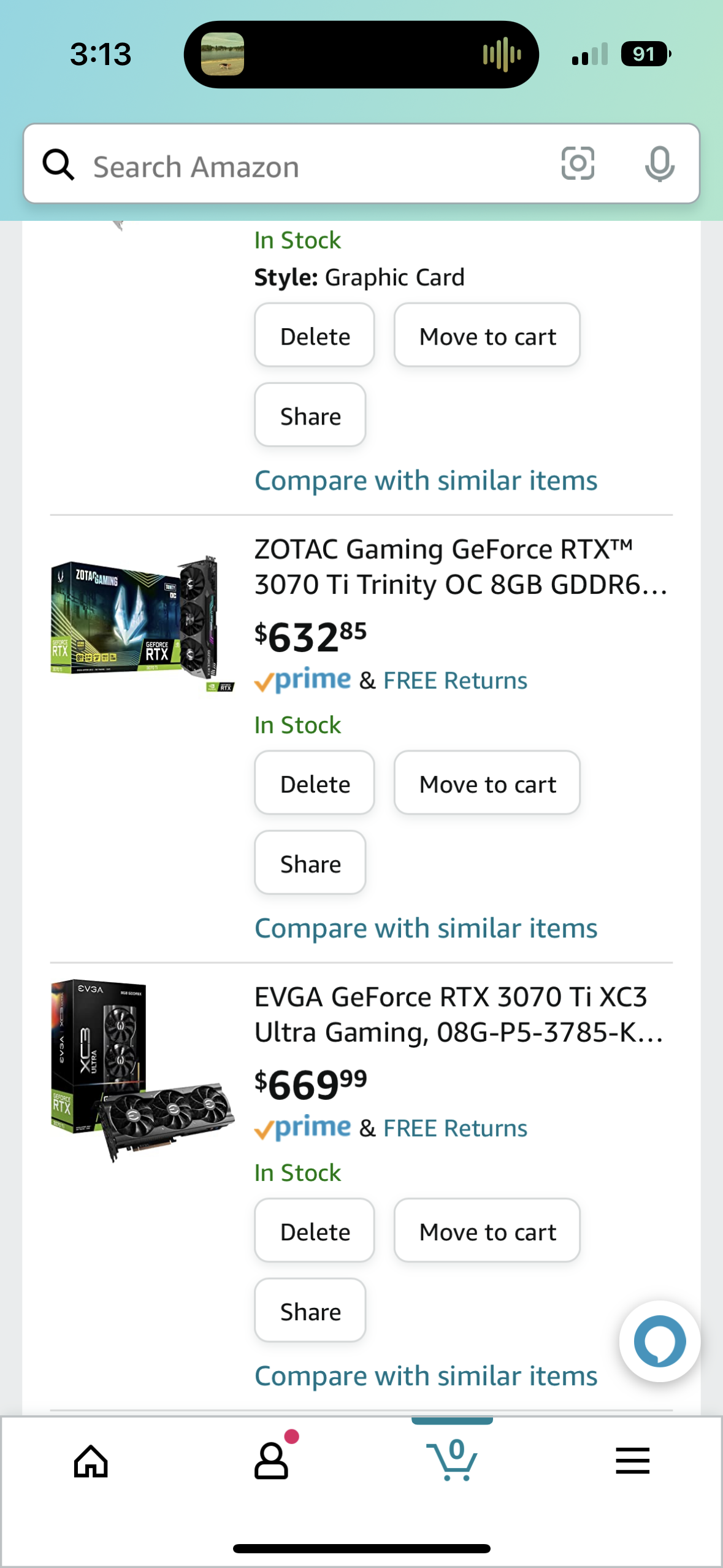In this detailed image screenshot, the status bar of a smartphone is clearly visible at the top. On the top left corner, the current time is displayed as 3:13. The top right corner showcases the network signal strength and the phone's battery level, which is at 91%. Centrally at the top, the dynamic island feature is also present. 

The main content of the screenshot is an Amazon webpage, which displays items in a card layout. Among the highlighted items are graphics cards. The first card features the Zotac Gaming GeForce RTX 3070 Ti Trinity Overclocked with 8GB GDDR6 memory, priced at $632.85. The third card in view shows the EVGA GeForce RTX 3070 Ti FTW3 Ultra Gaming model 08G-P5-3785, valued at $669.99.